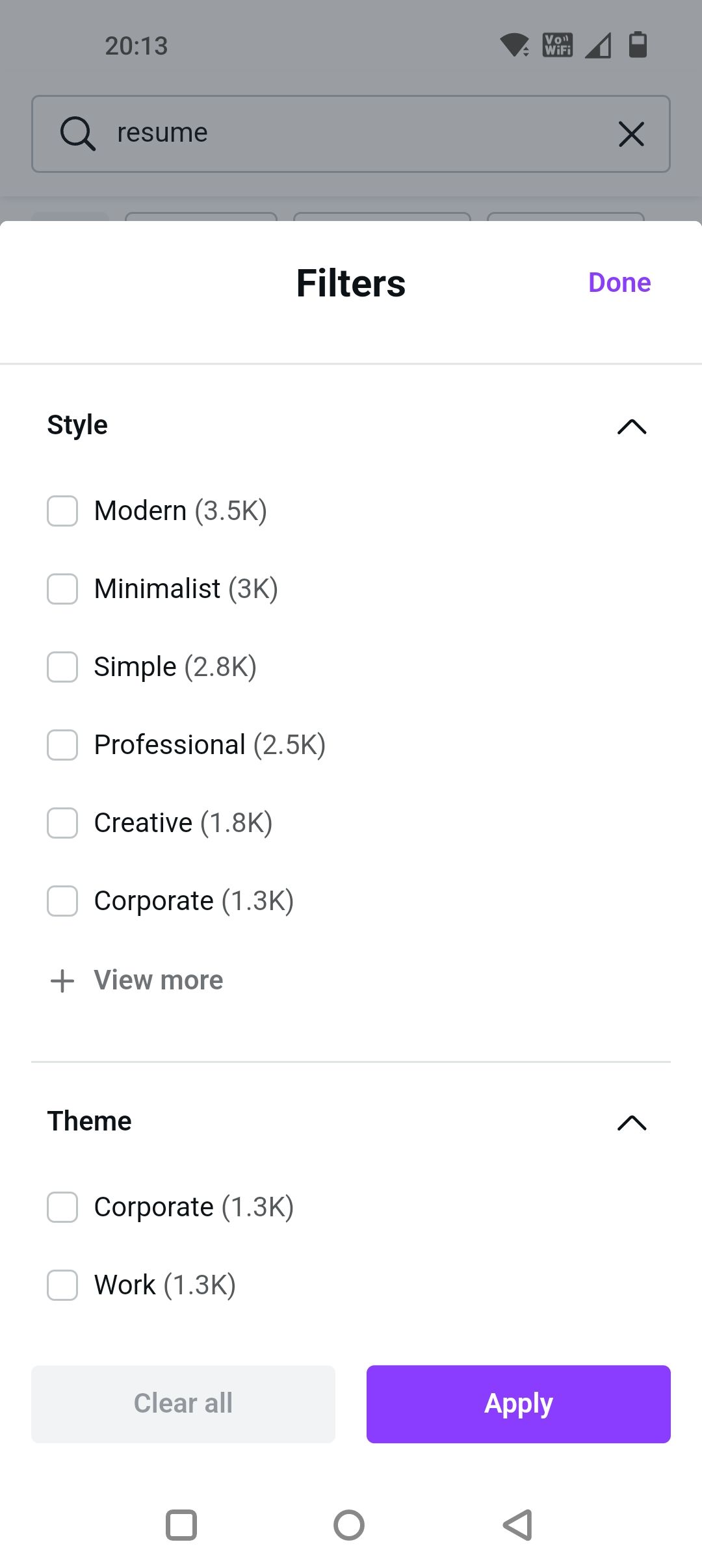This image is a screenshot of a website captured on an Android mobile device, with key interface elements indicative of its time being around 2013. The device status bar displays a partially filled cellular signal with about one-third strength, absence of a Wi-Fi connection, and approximately 50% battery life remaining. The screenshot prominently features a search bar at the top center, labeled “Resume” with a magnifying glass icon on the left and an 'X' icon on the right side, hinting at a search functionality related to resumes.

In the foreground, a pop-up window is visible, offering filter options for resume styles. The header of this pop-up reads "Filters" in bold black text, with the word "Done" in smaller purple text to finalize the selection. The filter options are laid out in a list format, allowing users to select one or multiple styles. The available resume styles listed include:
- Modern: 3.5K
- Minimalist: 3K
- Simple: 2.8K
- Professional: 2.5K
- Creative: 1.8K
- Corporate: 1.3K

There's also a "View More" option for additional styles. At the bottom of the filter list are two choices: "Clear all filters" or "Apply filters," giving the user control to reset or apply their selected filters respectively.

Judging by the interface and functionalities, this appears to be a resume template builder, designed to help users customize and optimize their resumes by choosing from various professionally designed styles.